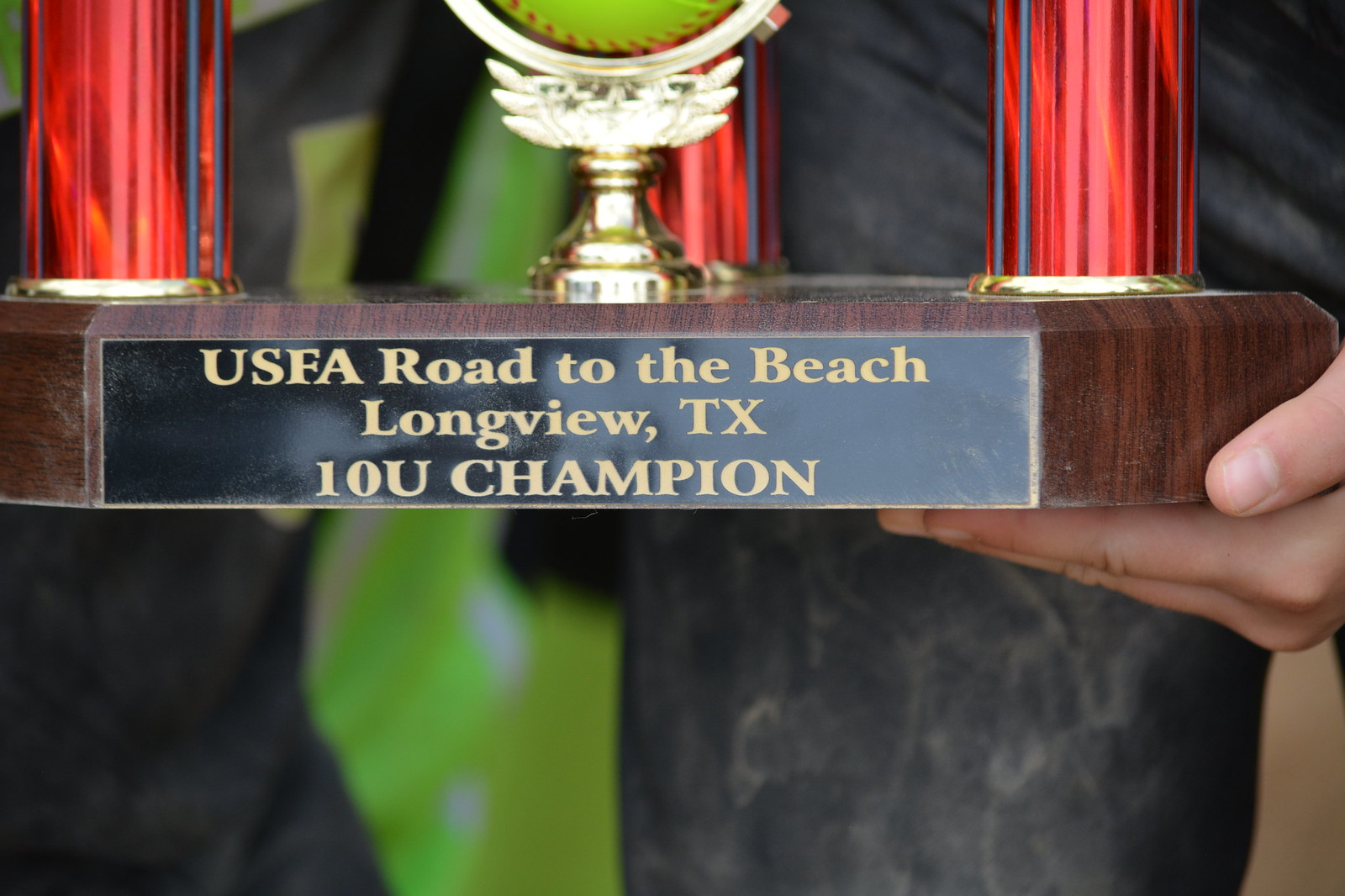In this close-up photograph, we see a trophy being held by a hand that enters the frame from the right side, with only the thumb and fingers visible. The focus of the image is the black placard on the wooden base of the trophy, which features gold engraving that reads, "USFA Road to the Beach, Longview, Texas, 10U CHAMPION." The trophy also includes red metallic columns and a gold centerpiece with wings, along with the bottom half of a green softball with red stitching. The blurred background, making it difficult to discern specific details, contains black and green hues, possibly indicating someone's clothing. The image appears to have been taken during an award presentation, though the exact setting and time of day remain unclear.